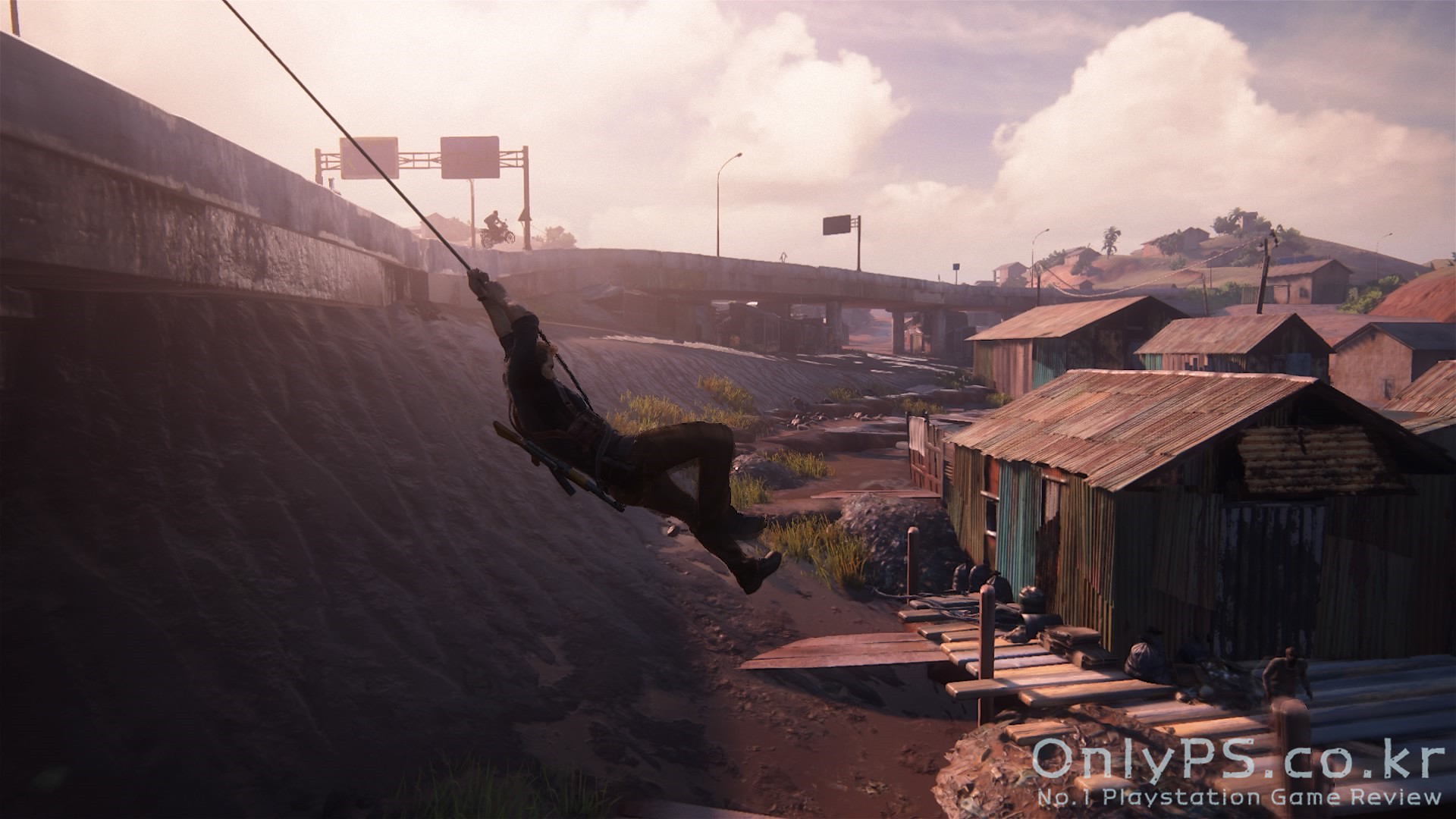In this hyper-realistic computer game still, the scene depicts a post-apocalyptic or war-torn area with a series of wooden shacks and sheds built below a roadway. A figure dressed in all black and wearing black boots is attached to a rope, swinging down from the elevated roadway on the left towards the shacks. The shacks are made of weathered wood with corrugated metal roofs and are supported on stilts above a dirt ground. Sparse greenery can be seen among the dirt, and patches of tall grass are scattered across the area. In the background, a roadway on an overpass zigzags across the image, with a person on a bike or motorcycle elevated in the air. Beyond the roadway, the landscape includes hills with trees and a sky filled with large white clouds. In the bottom right corner, the text reads "only ps.co.kr NO1 PlayStation Game Review."